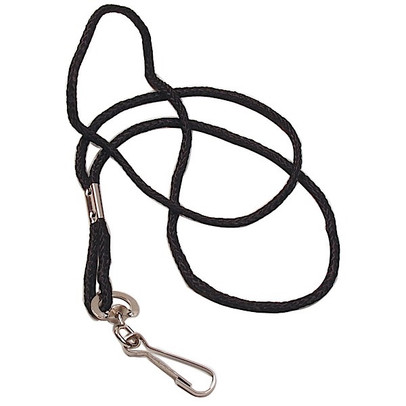The image features a black, woven or braided safety rope. It is somewhat tangled and laid out on a stark white background. The rope includes multiple metallic attachments: a silver clasp that secures the two ends of the rope, forming a smaller loop at the top, and another silver clasp that attaches to a silver carabiner. This carabiner is designed to clip onto items such as keys, ID tags, or potentially anything else that can be looped through and held securely. Despite some initial ambiguity about its use, the combination of its design elements and the materials suggest it is more likely a lanyard or name tag holder rather than a dog leash, given its apparent length and strength.